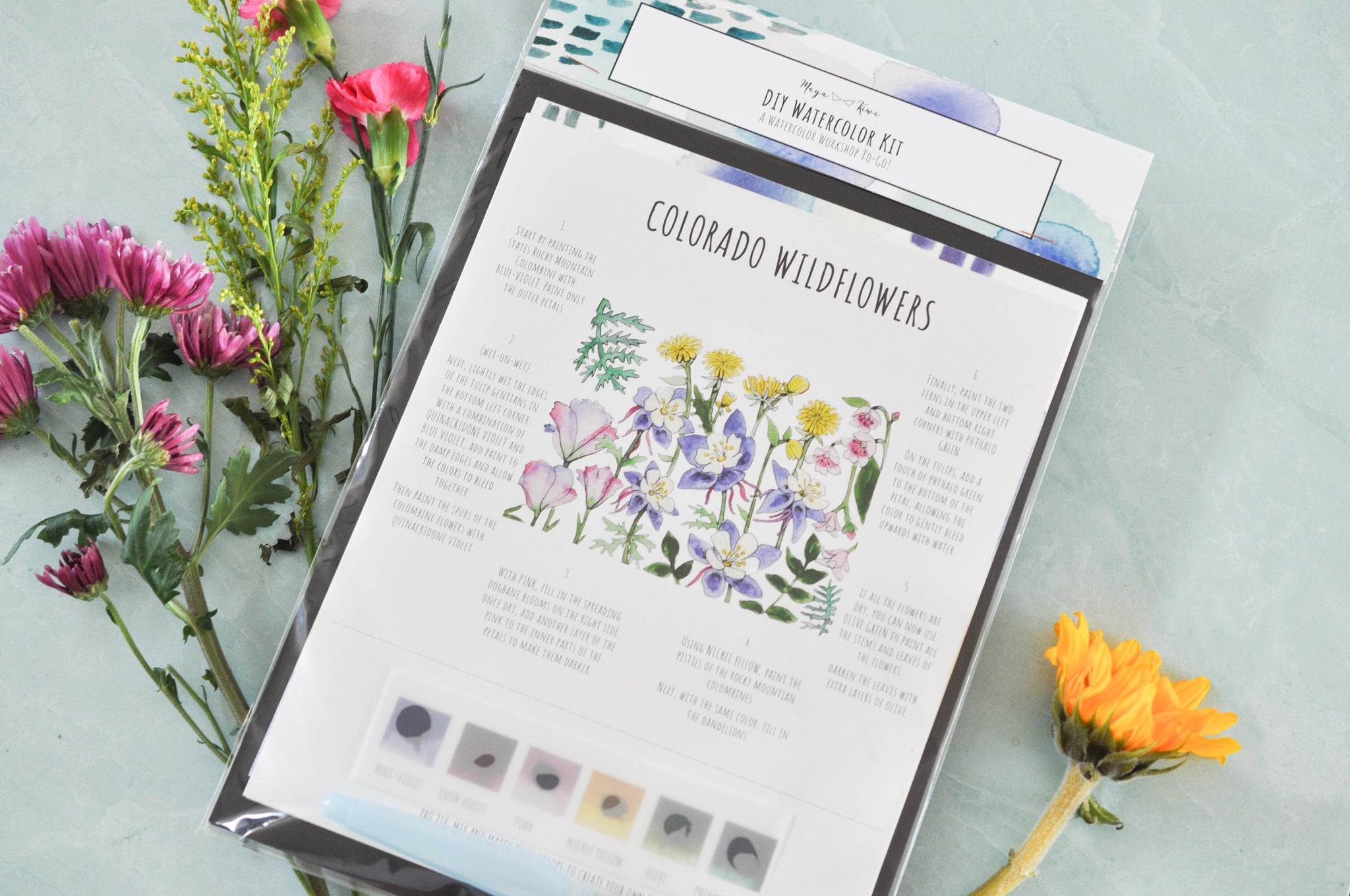This image features a DIY Watercolor Kit lying on a marble-like light blue countertop. The white card, slightly tilted to the right, prominently displays "DIY Watercolor Kit" at the top in black text. Directly below that, the text "Colorado Wildflowers" is also in bold black letters. In the center of the card, an illustrated diagram showcases various wildflowers in hues of yellow, purple, pink, and white, with detailed text in thin black lettering encircling the diagram. To the bottom right corner of the card, a yellow flower, possibly a daffodil or dandelion, is visible, while to the left corner, there is a cluster of wildflowers with green stems and pinkish-purple blooms. Additional floral elements, including a yellow daisy and violets on green stems, enhance the natural, colorful theme of the DIY Watercolor Kit displayed on this delicately set package.